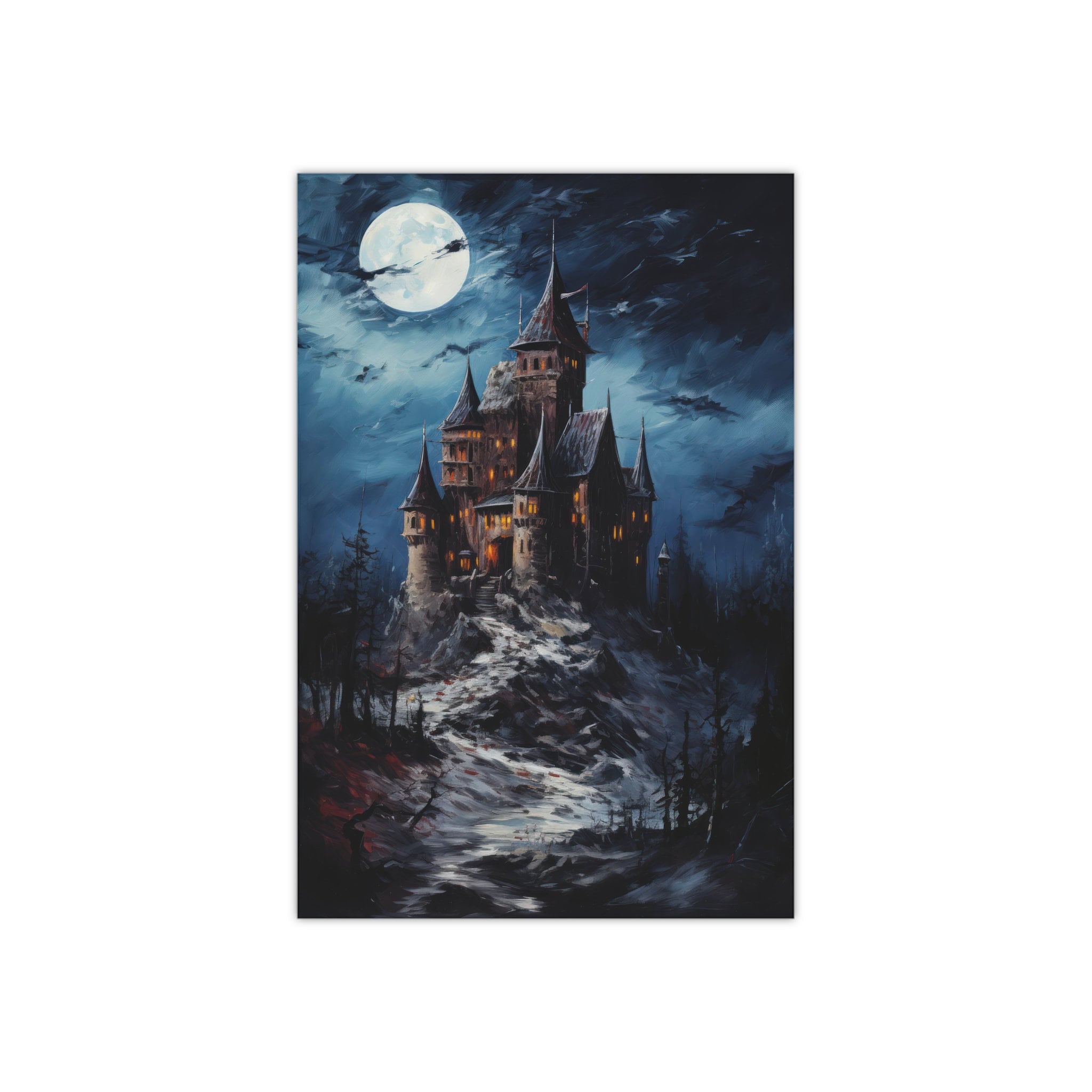This detailed color illustration depicts a towering, ominous castle situated on a rugged, snowy hill. The castle, rendered in shades of brown and rusty blue, features numerous tall turrets adorned with spiky tops and lit windows emitting an eerie orange glow. Surrounding the castle, sharp stones and dead trees contribute to the foreboding atmosphere. The dark, stormy sky dominates the scene, with turbulent clouds and a full moon illuminating the top left corner. Bats can be seen flying around the moon, adding a spooky element. A winding, rocky pathway, distinctly lit by the moonlight, leads up to the imposing castle, creating a vivid and chilling scene.